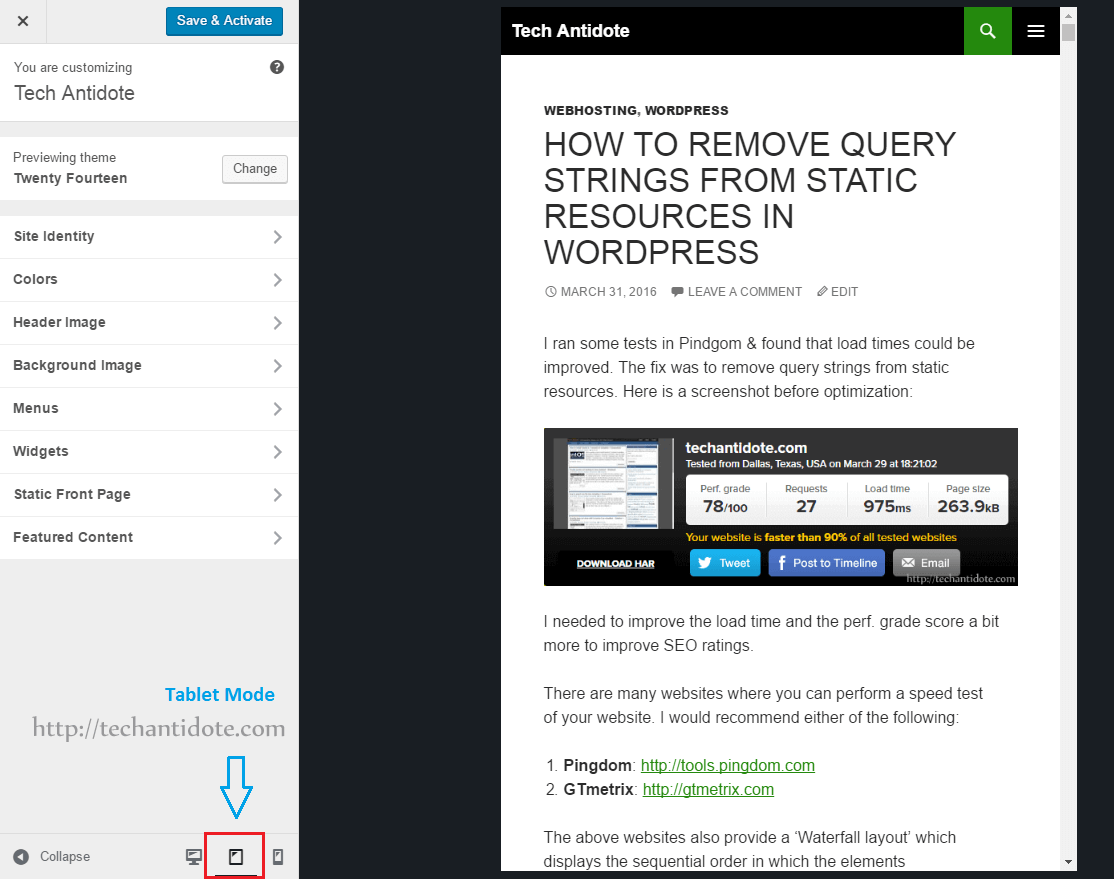The screenshot showcases a user interface for customizing a web theme. On the left side, there is a vertical white rectangle, while the rest of the background is black. At the top-left corner sits a light gray rectangle featuring a black "X" button. Adjacent to this, on the right, is a blue button labeled "Save & Activate". Below this, in smaller gray text, it reads "You are customizing", followed by larger gray letters that spell "Tech Antidote".

In the upper right-hand corner, there is a black circle with a white question mark inside. Beneath this lies a thick horizontal gray line. Below this line, the text "Previewing Theme" appears in gray, followed by the bolded text "2014". To the far right, there is a gray "Change" button. Another thick gray horizontal line follows.

Below these lines, there is a menu of items each with right-pointing arrows resembling gray sideways "V" shapes. These items are bolded in black and include:
- Site Identity
- Colors
- Header Image
- Background Image
- Menus
- Widgets
- Static Front Page
- Featured Content

Further down, the left side of a gray square is visible. At its center in blue text, it says "Tablet Mode". Below, part of a website address and the outline of a downward-pointing blue arrow are visible.

On the right side, the top section displays "Tech Antidote" in white text. Adjacent to it is a large white rectangle. At the top of this rectangle, in bold black text, it reads "Web Hosting, WordPress". Below this, in large black letters, it states "How to Remove Query Strings from Static Resources in WordPress". Following this title is a paragraph, and within it, there's a black rectangle containing tech-related information, followed by more text.